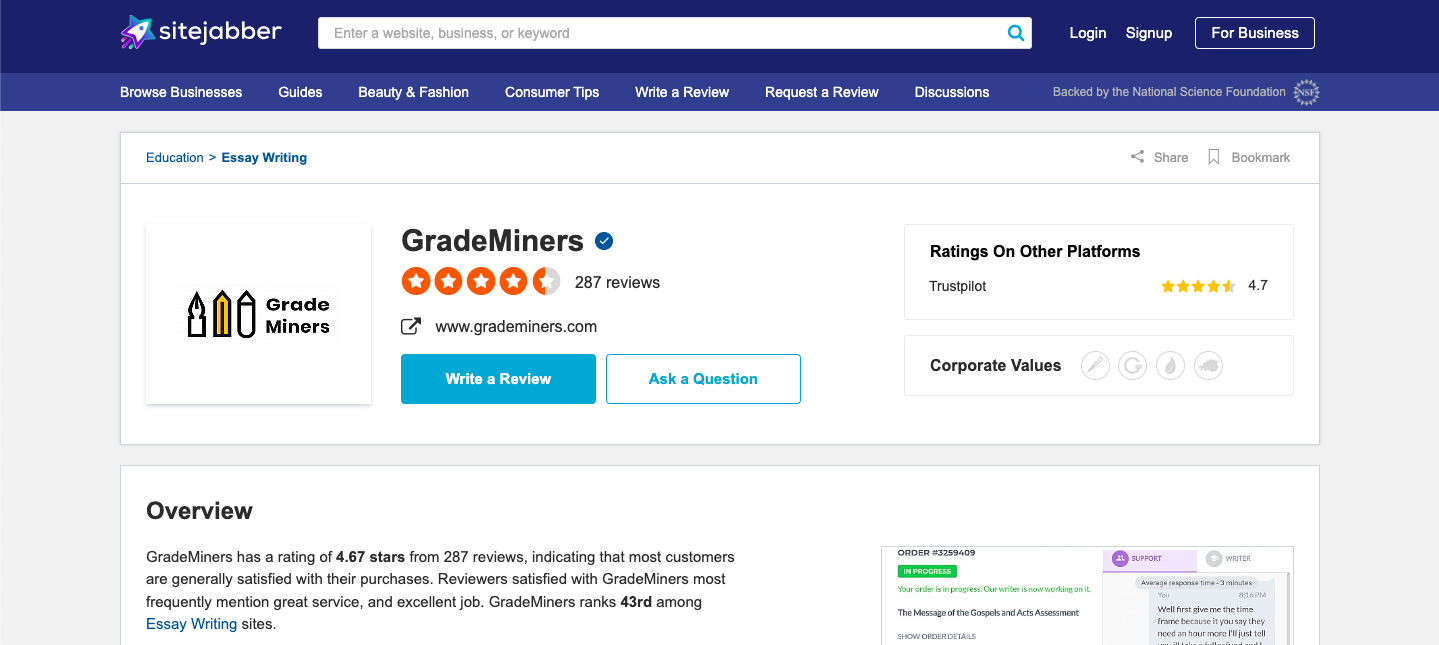The image is a screen capture of the SightJabber website displayed on a computer monitor. 

At the very top, a dark blue banner—almost black on the left side—spans across the width of the screen. Positioned to the left on this banner is a logo featuring a green, blue, and purple star designed to resemble a rocket. To the right of the logo, the site name "SightJabber" is rendered in lowercase white text. 

Center-top is a streamlined white search bar featuring a turquoise magnifying glass icon on its right end. Adjacent to the search bar, from left to right, are options in white text for "login," "sign up," and a white-outlined button labeled "for business."

Below this, a lighter blue horizontal bar holds various site navigation options in white text, listed from left to right as: "browse businesses," "guides," "beauty and fashion," "consumer tips," "write a review," "request a review," "discussions," and a note indicating the site is "backed by the National Science Foundation," accompanied by their logo on the far right.

Central to the image, the main content area is enclosed in a rectangular white section. On the upper left in blue lettering, the category "education" is listed, followed by a forward arrow and "essay writing." The upper right section displays a share icon and a bookmark icon.

Prominently featured in the center is the name "Grade Miners" in bold black text, accompanied by a blue circle containing a white check mark. The adjacent rating shows four and a half orange stars based on 287 reviews. Directly beneath the name, the URL for Grade Miners is presented in black text. A large blue button on the left, labeled “write a review,” contrasts with a white “ask a question” button with blue text on the right.

To the left, three icons—a pen, a pencil, and an eraser—are displayed. On the right, there's a section labeled “ratings on other platforms” featuring a Trustpilot rating of 4.7, along with icons linking to corporate values.

At the bottom left, the word "overview" appears in bold black, with a descriptive paragraph about Grade Miners' ratings beneath it. In the bottom right corner are two small boxes; the left one is green with black text showing an order number and a green “in progress” button. The right box is purple and features a lavender-colored "submit" button.